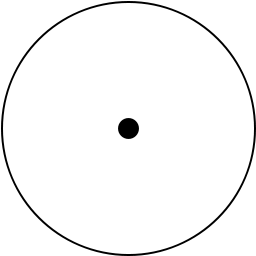This is an image featuring a minimalist geometric design, devoid of any background or framing. At the center of this design is a black circle with a solid black dot precisely in the middle. The circle's outline appears slightly pixelated, indicating a lower resolution, suggesting it could be created with almost any basic graphics software, such as Microsoft Word, Excel, or even more advanced programs like Photoshop or Illustrator. The stroke of the circle is relatively narrow, while the central dot is somewhat larger, giving the overall impression of an eyeball viewed from above. The image offers no additional context, leaving its purpose or symbolism open to interpretation.